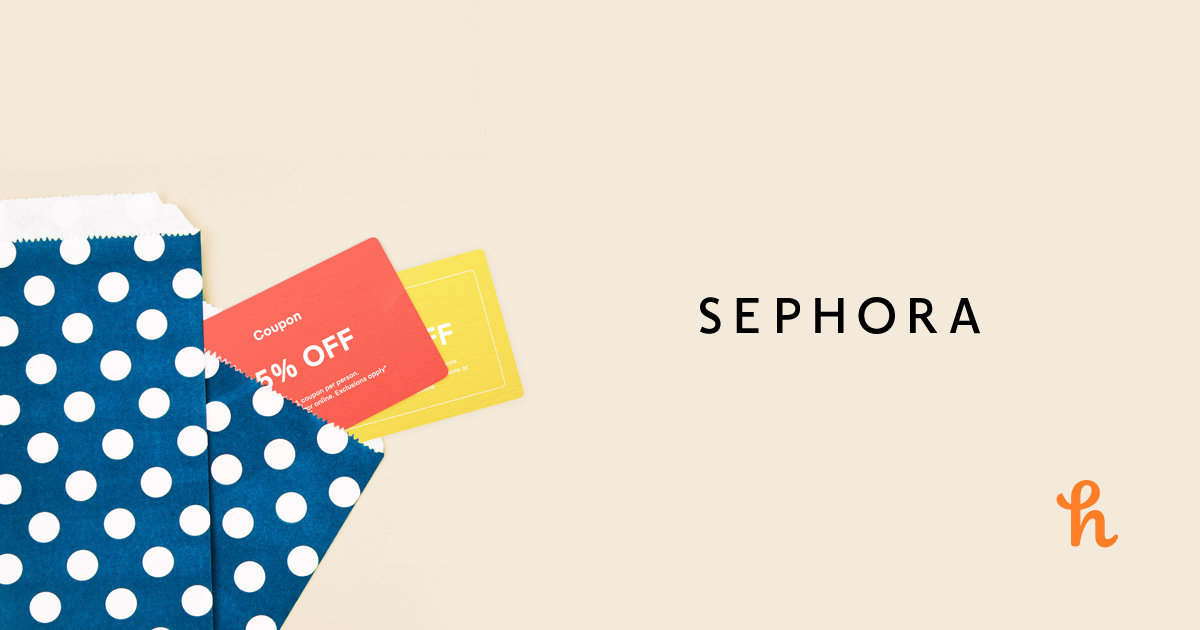A detailed and descriptive caption for the image would be:

"The image is a rectangular, landscape-oriented screenshot set against a beige background. Dominating the center of the image is the word 'SEPHORA' in bold, black capital letters. In the bottom left-hand corner, there is an orange, cursive lowercase 'h'. Adjacent to this, also in the bottom left, are two navy paper bags adorned with white polka dots. The first bag is partially behind the second one, which is tilted at an angle, leaning to the right. Protruding from the top of these bags are two cards. The front card is red and partially inserted into the bag, displaying the words 'coupon' and '5% off' in white text; however, part of the text is obscured due to the cropping. Behind it, a yellow card is visible, displaying a partially recognizable letter 'F'. The simplicity and clean design of the image are accentuated by the unembellished beige background."